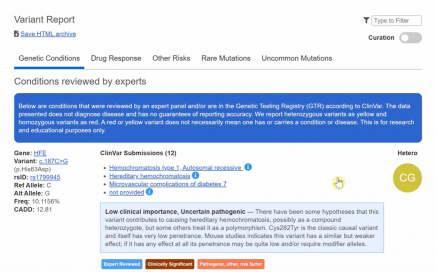The image is a rectangular screenshot of a website featuring a predominantly white background. The top left corner displays the title "Variant Report" in black text, and directly below it, the option "Save HTML Archive" in blue text. In the top right corner, there is a search bar with a filter icon shaped like an elongated hourglass. Inside the search bar, the placeholder text reads "Type to Filter" in gray.

Below the search bar, the heading "Curation" appears in black text, accompanied by an oval-shaped toggle button that is gray with a white circle positioned on the left side, indicating that it is turned off.

Further down, the page is segmented into several clickable options listed in black text: "Genetic Conditions," "Drug Response," "Other Risks," "Rare Mutations," and "Uncommon Mutations." These options are arranged from left to right.

Following these options, there is a section titled "Conditions Reviewed by Experts." Below this heading, a blue rectangular box with white text and rounded corners provides additional information. The text begins with "Below are conditions that were reviewed by an expert panel and/or are in the Genetic Testing Registry (GTR) according to ClinMax. The data presented does not diagnose disease and has no guarantees of reporting accuracy. Re-report..." The text appears to continue beyond what is visible.

This descriptive caption offers a clear and detailed overview of the website's layout and contents as depicted in the screenshot.